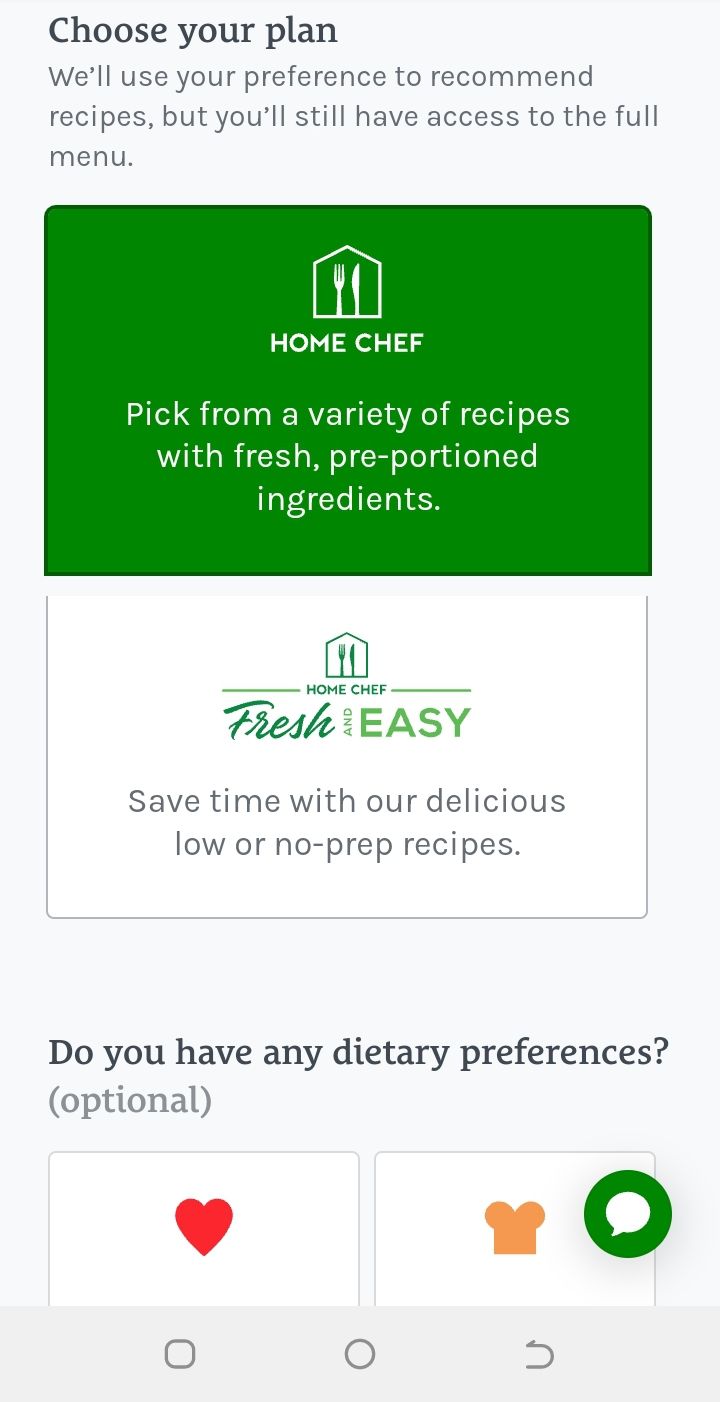This image is a screenshot captured from a digital device, possibly a laptop, desktop, tablet, or smartphone. The screen features a mid-grey background with bold black text at the top that reads "Choose Your Plan." Beneath this text is another message in black that states, "We'll use your preference to recommend recipes, but you still have access to the full menu." 

Central to the image is a dark green rectangle containing a white house-like emblem with a fork and knife, signifying the "Home Chef" service. Below this emblem, in bold white text, it reads "Home Chef," and further down in regular white text, it mentions, "Pick from a variety of recipes with fresh, pre-portioned ingredients."

Adjacent to this is a white rectangle adorned with a similar emblem; however, this time, the house symbol along with the fork and knife is dark green. "Home Chef" is written in dark green at the bottom, accompanied by lime green borders on the left and right sides. In cursive dark green text, the word "fresh" is displayed, followed by "and" in lime green, with "turn sideways" appearing to clarify that the text orientation is flipped. The caption in black reads, "Save time with our delicious low or no-prep recipes."

Further down, a bold black question arises, "Do you have any dietary preferences?" followed by an optional note in grey parentheses. Below this, there are two selectable options represented by squares: the first is white with a red heart symbol, and the second is brown, resembling a loaf of bread. Lastly, there's a dark green chat symbol—a circle with a white inner circle and a bezel at the bottom displaying a dark grey square, circle, and back symbol.